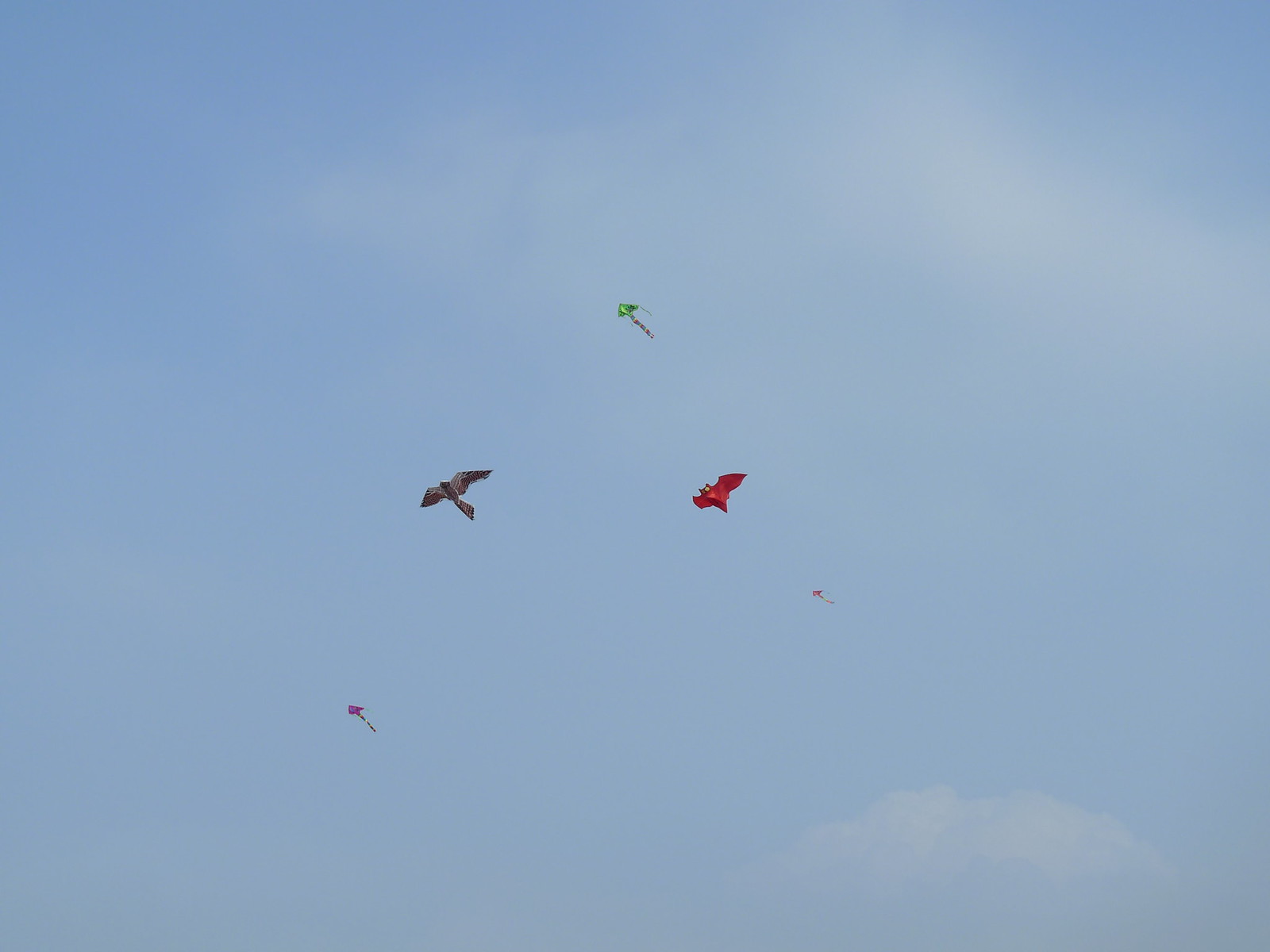The image captures a tranquil scene of five kites soaring high in a muted blue sky with faint, wispy white clouds. Two kites, a red one resembling a bat and a black one shaped like a bird, are prominently featured in the middle, closer to the foreground. Higher up in the sky is a bright green kite, while two smaller kites, whose colors appear to be red and are much further away, complete the scene. All the kites are gliding towards the left, suggesting they are part of a leisurely event or family outing. Despite the clear day, the photo lacks vibrant contrast, giving it a soft and subdued aesthetic. No visible strings anchor the kites, leaving them to appear effortlessly adrift against the expansive sky.